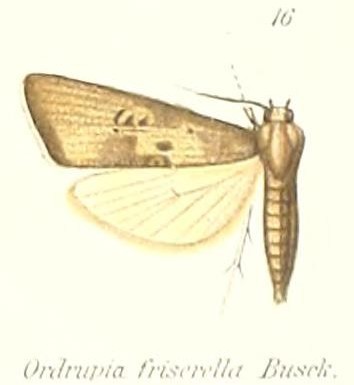This image is a detailed color illustration of a moth, presented in a square format with a slightly taller height than width. The background is a cream color, lending a vintage or guidebook quality to the illustration. The focal point, positioned centrally, is the moth, drawn with its body oriented vertically on the right side of the image and its wings spread to the left. The moth’s body and the upper part of its left wing are a dark brown color, with the wing featuring circular dots adding intricate detail. The lower part of the left wing transitions to a lighter cream color with beige veins. Only one of the moth’s antennae is visible, located on the top left of its head, along with two small eyes. The number 16 appears in green text near the upper right corner of the image. Along the bottom edge, there is a line of text, possibly in another language, which reads "Ardrupia friscarella brusque" in a light gray font. This blend of detailed illustration and typography captures the essence of a scientific or educational depiction of the insect.